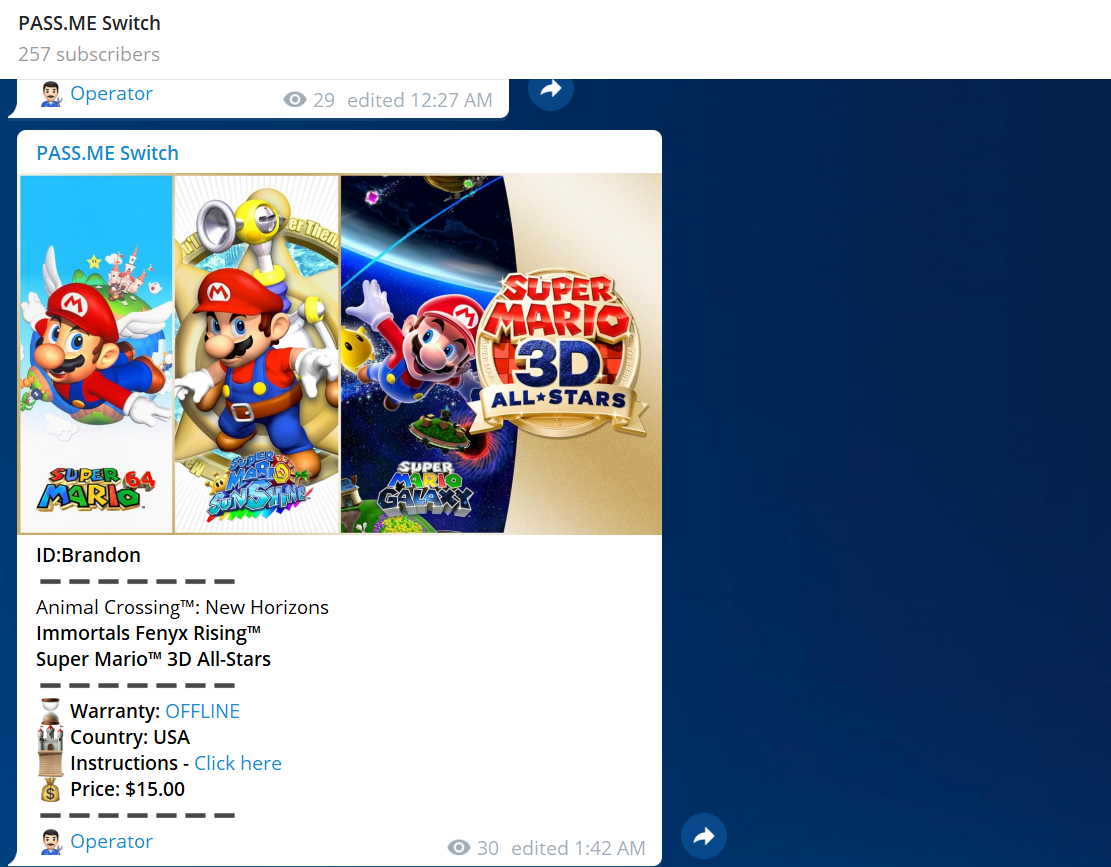This is a detailed caption for an image taken from a Super Mario Brothers game interface:

The image is a screenshot from a Super Mario Brothers game interface. At the top of the interface, there is a text that reads "pass emmyswitch," followed by the number of subscribers, "257 subscribers." Below this, there is a bar showing the label "operator" accompanied by a small icon of a person, the number "29," and the text "edited, 12:27 a.m."

The background of the interface features a large purple-blue box, while a prominent white pop-up box overlays it, containing key information. The pop-up box prominently displays the text "pass me switch." Inside this box, there are three images of Mario from the game:

1. The first image shows Mario with the label "Super Mario 64."
2. The second image depicts Mario standing.
3. The third image shows Mario in space with the label "Super Mario 3D All-Stars."

Further details under the images list:
- An ID: "Brandon,"
- Video games: "Animal Crossing: New Horizons," "Immortals Fenyx Rising," and "Super Mario 3D All-Stars."
 
Below this section, additional information is displayed, including:
- "Warranty: Offline,"
- "Country: USA,"
- A prompt for instructions: "Click here,"
- The price: "$15."

An operator button with a human icon is situated at the bottom, followed by the numbers "30 edited" and "1:42 a.m." There is also a small blue button with an arrow next to it, positioned adjacent to the operator section.